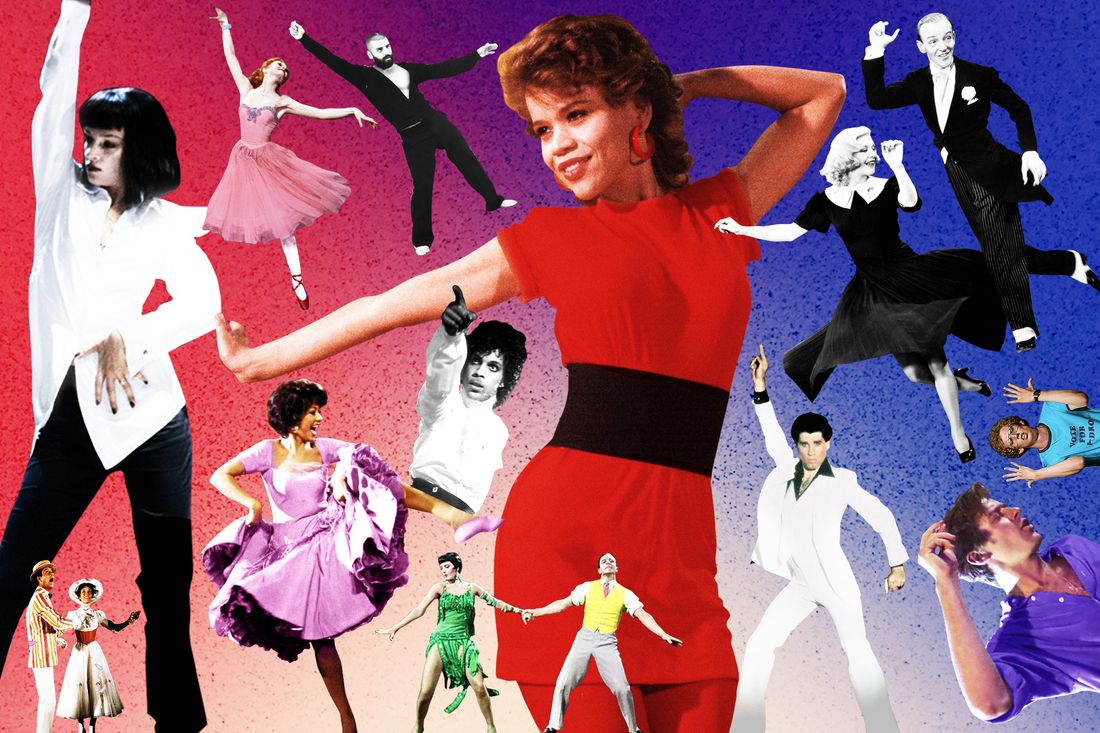This vibrant collage features an array of famous celebrities captured in iconic dance poses, set against a dynamic background that transitions from pink to purple to blue. Central to the image is a woman in a striking red outfit, smiling to the side. Surrounding her are silhouettes and full-color depictions of well-known figures such as John Travolta in his iconic white suit from "Saturday Night Fever" striking a disco pose, Prince with his signature poofy hair and black gloves pointing dramatically, and Uma Thurman's character from "Pulp Fiction" in a white dress shirt and black bell-bottom pants. Also included are Fred Astaire, Mary Poppins, and the character from "Napoleon Dynamite" performing his memorable talent show dance. The scene exudes a vintage, retro vibe, with the celebrities outfitted in traditional, era-specific costumes, celebrating the timeless art of dance and choreography.